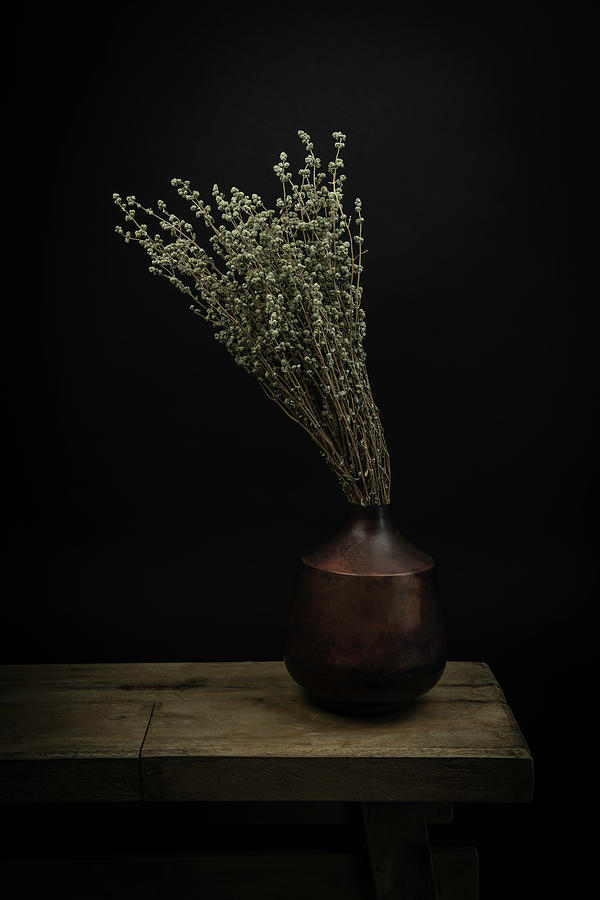In this striking still life photograph, the centerpiece is a rustic brown vase with a squat, rounded base that narrows into a narrow neck. It appears to be made of dark wood or possibly repurposed copper, exuding a DIY and rustic charm. The vase is filled with a bouquet of dried plant stalks, which resemble twigs or perhaps dried baby's breath, complete with very small white flowers. These stalks, standing twice the height of the vase, lean slightly to the left, adding a dynamic touch to the composition. This arrangement sits on the right-hand side of what looks like an unfinished wooden bench or rustic table, cropped on the left side. The backdrop is a solid black wall, emphasizing the still life through stark contrast. The lighting is dark, creating a dramatic, minimalist setting that highlights the textures and forms within the image.